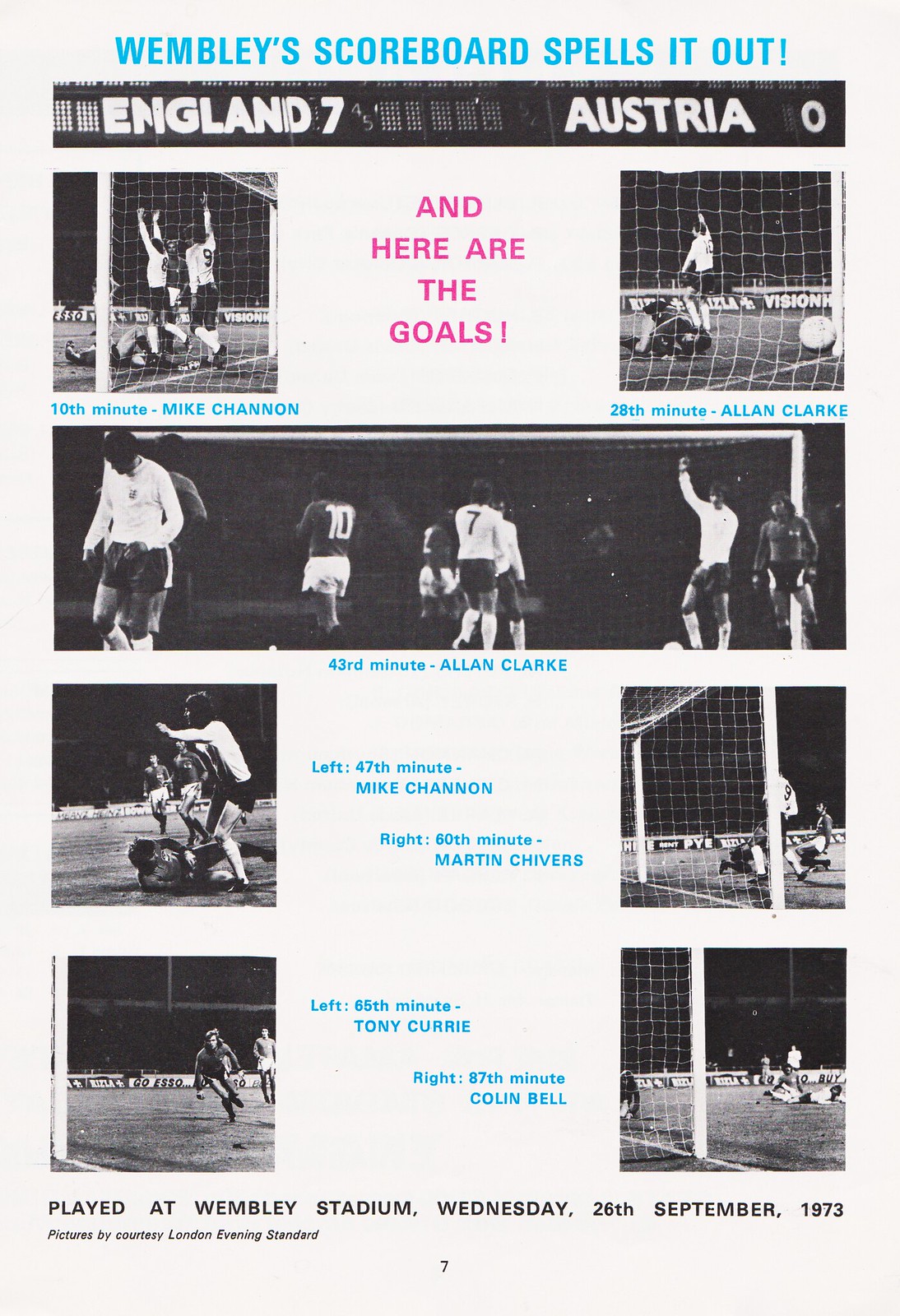The image is a detailed poster showcasing the events of a soccer match played at Wembley Stadium on Wednesday, 26 September 1973. At the top of the poster, in a blueprint uppercase font, it declares "Wembley's scorecard spells it out." Below this, on a black horizontal border in white uppercase font, it prominently displays the score "England 7 Austria 0." Centered beneath this, in uppercase red font, the poster announces "AND HERE ARE THE GOALS." The main section features seven black and white photographs illustrating key moments from the game, each accompanied by blue text detailing the minute and the player who scored: 10th minute - Mike Shannon, 28th and 43rd minutes - Alan Clark, 47th minute - Mike Shannon, 60th minute - Martin Chivers, 65th minute - Tony Curry, and 87th minute - Colin Bell. The layout includes two photos at the top (left and right), a large central image, followed by two more photos positioned on the left and two on the right, showcasing various in-game actions and players interacting with the soccer nets. At the bottom of the poster, in black uppercase font, the details "Played at Wembley Stadium Wednesday 26 September 1973" are reiterated.